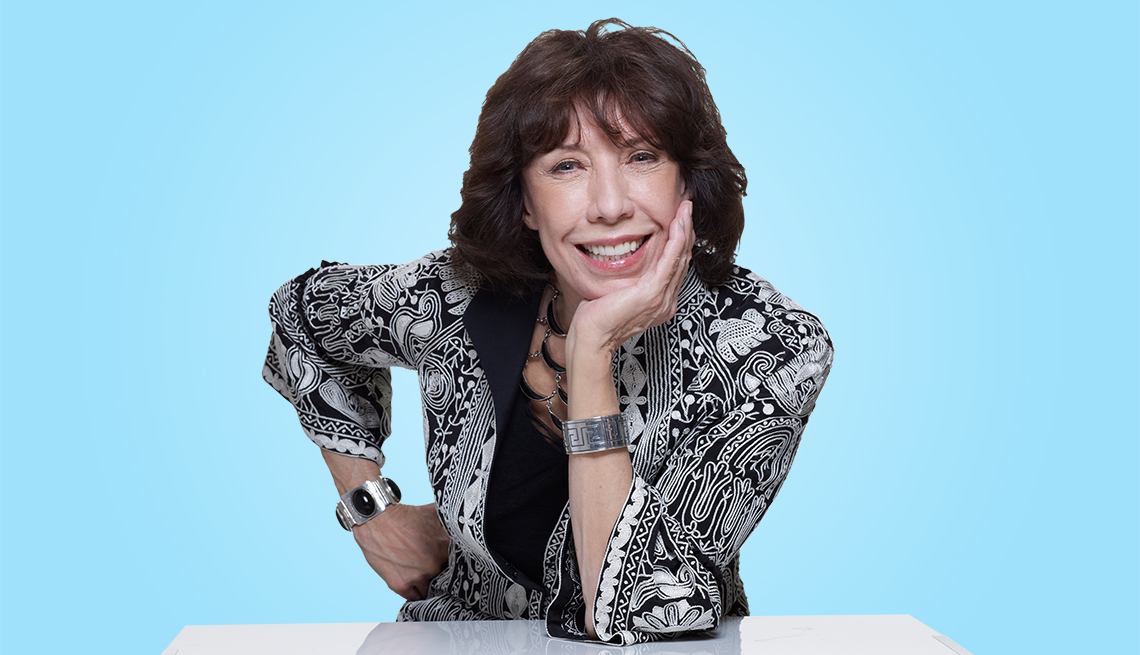In this professional headshot, an older woman, likely in her 60s, is depicted against a vivid blue background. She has dark brown hair that reaches her shoulders, styled with bangs and soft waves. Smiling warmly, her face is gently cupped in her left hand, with her elbow resting on a sleek white table. Her right hand rests on her hip, forming a clenched fist. She wears a distinctive black jacket adorned with various white functional designs and patterns. Accessorizing her look, she has a chunky necklace around her neck and is adorned with silver bracelets on both wrists. The bracelet on her right wrist features a prominent black gem, while the one on her left displays intricate line designs and geometric shapes.